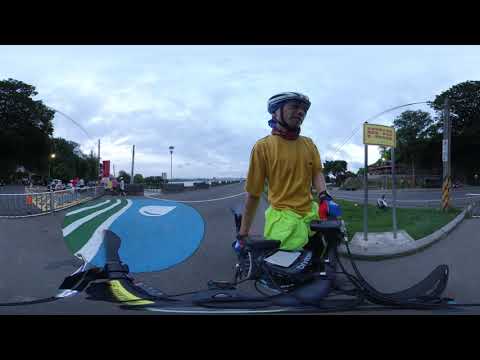In the image, there is a person standing outdoors on a cloudy day, positioned centrally. They are wearing a black and white helmet with large white spots or stripes, a mustard-colored shirt, fluorescent green shorts or pants, and blue and red gloves. A buff is wrapped around their neck. The person is standing beside their black bike, which has yellow handles, on a gray asphalt surface. To their left, there is a distinctive yellow, rectangular sign featuring a blue circle with a white water drop and green and white vertical lines. Trees frame the right and left edges of the image. The scene appears to be in a parking lot or similar open area, and the sky is overcast. A black border is present at both the top and bottom of the image. The setting is outdoors, during the day.